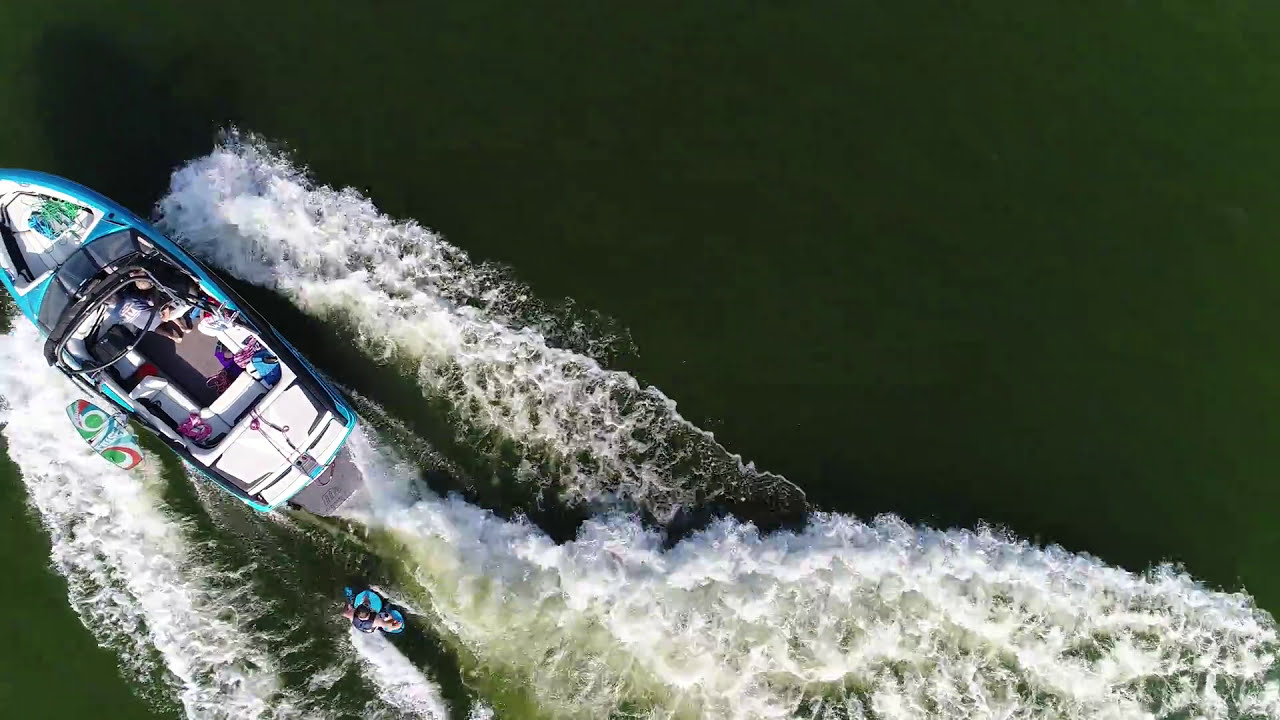This aerial image captures a dynamic scene of water sports on a large, green-tinted body of water. The focal point is a bright, neon blue and white speedboat, positioned to the far left of the frame. The boat is accented with a vivid green and red wakeboard hanging off its side. The boat's interior showcases a clean, white U-shaped seating arrangement. Trailing behind the boat is a wakeboarder, distinguishable by a blue life jacket and a blue wakeboard. The wakeboarder glides over churning white waves created by the boat, which surge across the bottom and right side of the image. The perspective emphasizes both the rapid motion and the enjoyment of the day spent boating and engaging in water sports activities.